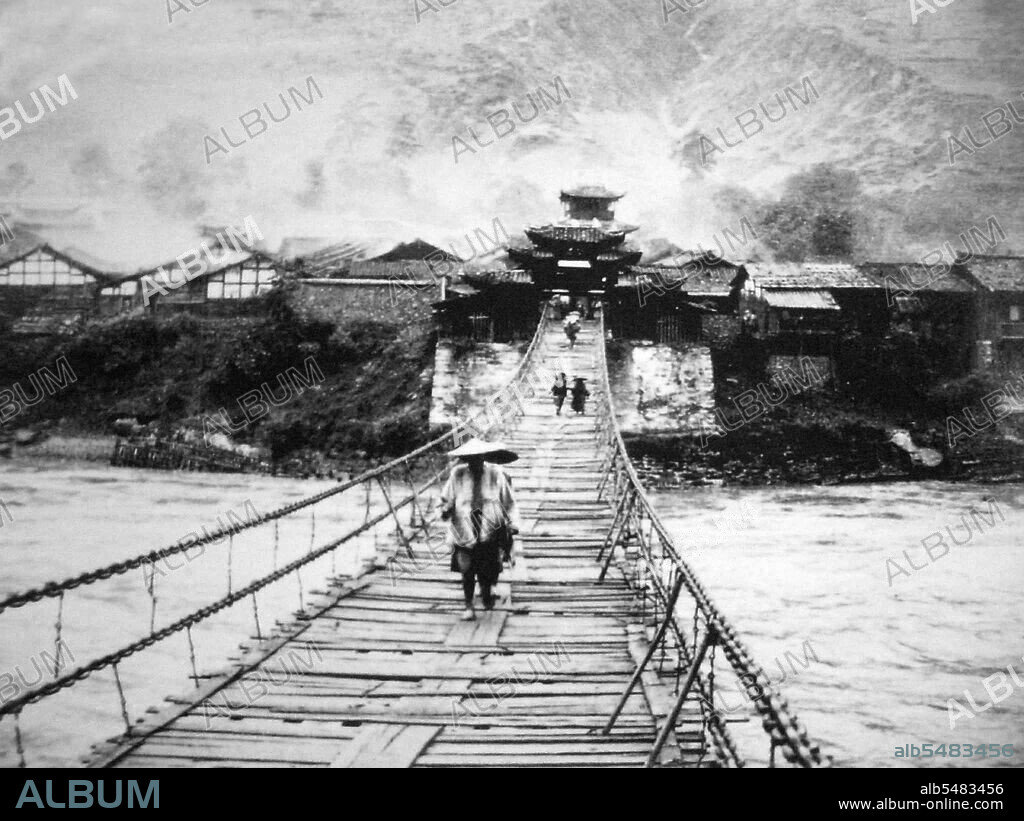This black-and-white photograph captures a long, wooden plank bridge with ropes or chains as railings, extending over a river. The bridge, appearing to be in an Asian country, leads towards a collection of Asian-style buildings, including a temple. A group of people is seen crossing the bridge, their expressions seemingly downtrodden, potentially due to the downcast and gray atmosphere of the image. One man close to the camera stands out, wearing a circular straw hat and light-colored attire. The sky above is gray, adding to the somber mood. The image is marked with watermarks reading "album" diagonally across, and the bottom edge includes a black bar displaying "ALB54834" on the left and "www.albumonline.com" on the right.